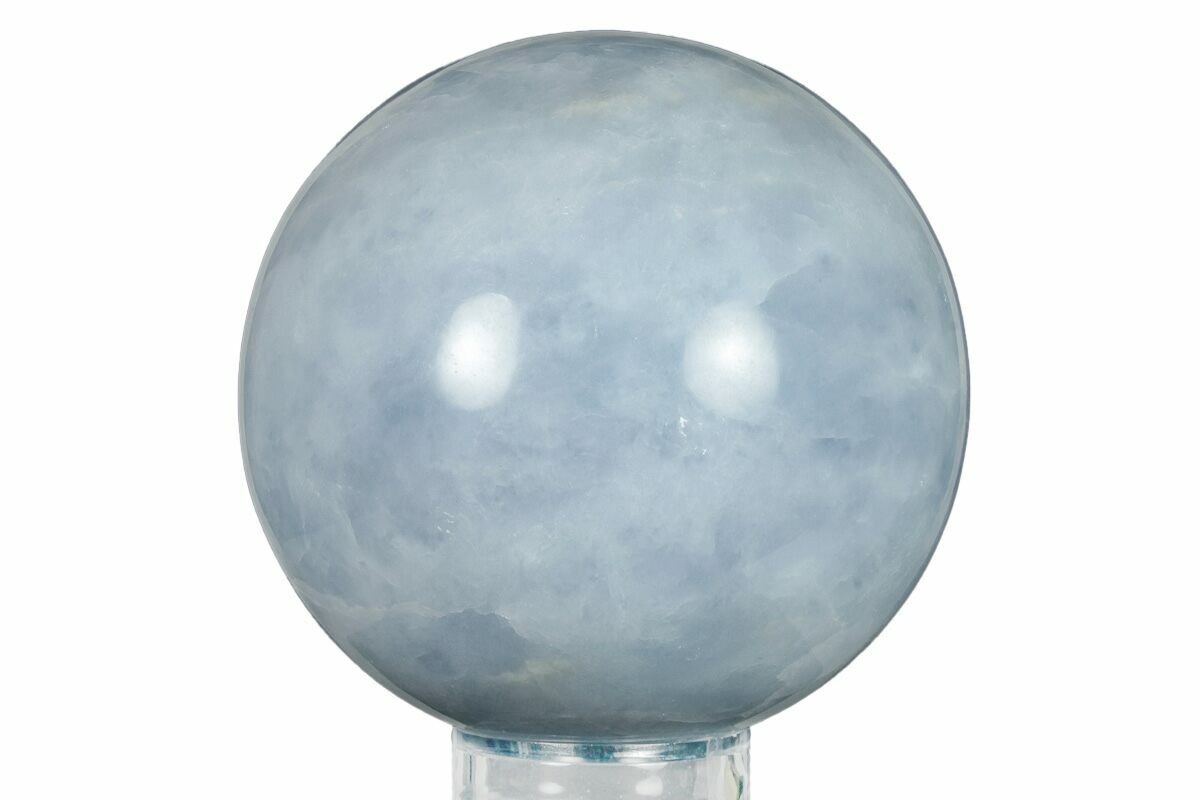The image depicts a glossy, round glass sphere with a swirling, smoky texture of light gray and bluish-gray hues, accented with subtle shades of off-blue and white. The sphere, approximately the size between a large marble and a small bowling ball, is seated on a sleek glass stand. The white background provides no additional context, suggesting the sphere may be featured for sale. The design includes two noticeable white glare spots, likely reflections, and the sphere exhibits a slightly marbled appearance, contributing to its intricate, cloudy interior pattern.